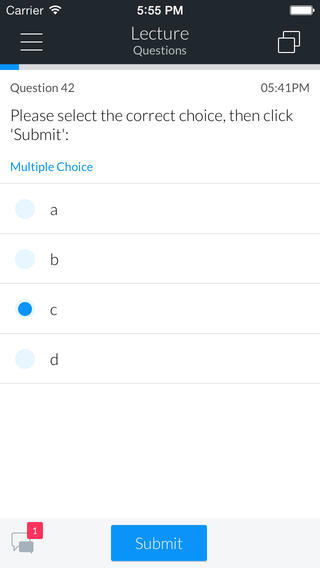This screenshot, captured from a mobile device, showcases a quiz-taking application interface. At the top of the screen, the status bar displays "Carrier" on the left, a full Wi-Fi signal, the current time "5:55 PM," and a fully charged battery icon on the right. The screen header reads "Lecture Questions," flanked by a menu icon on the left and a copy icon on the right. Beneath the header is a progress bar that is barely filled, indicating that the user has not completed much of the quiz. 

The interface shows that the user is on question 42, which they started at "5:41 PM." The instructions read, "Please select the correct choice, then click Submit," with "Multiple Choice" highlighted in blue text underneath. Four answer options labeled "A," "B," "C," and "D" are displayed, with option "C" selected. A prominent blue "Submit" button appears below the answer choices. The background of the page is predominantly white, providing a clear and uncluttered view of the quiz interface.